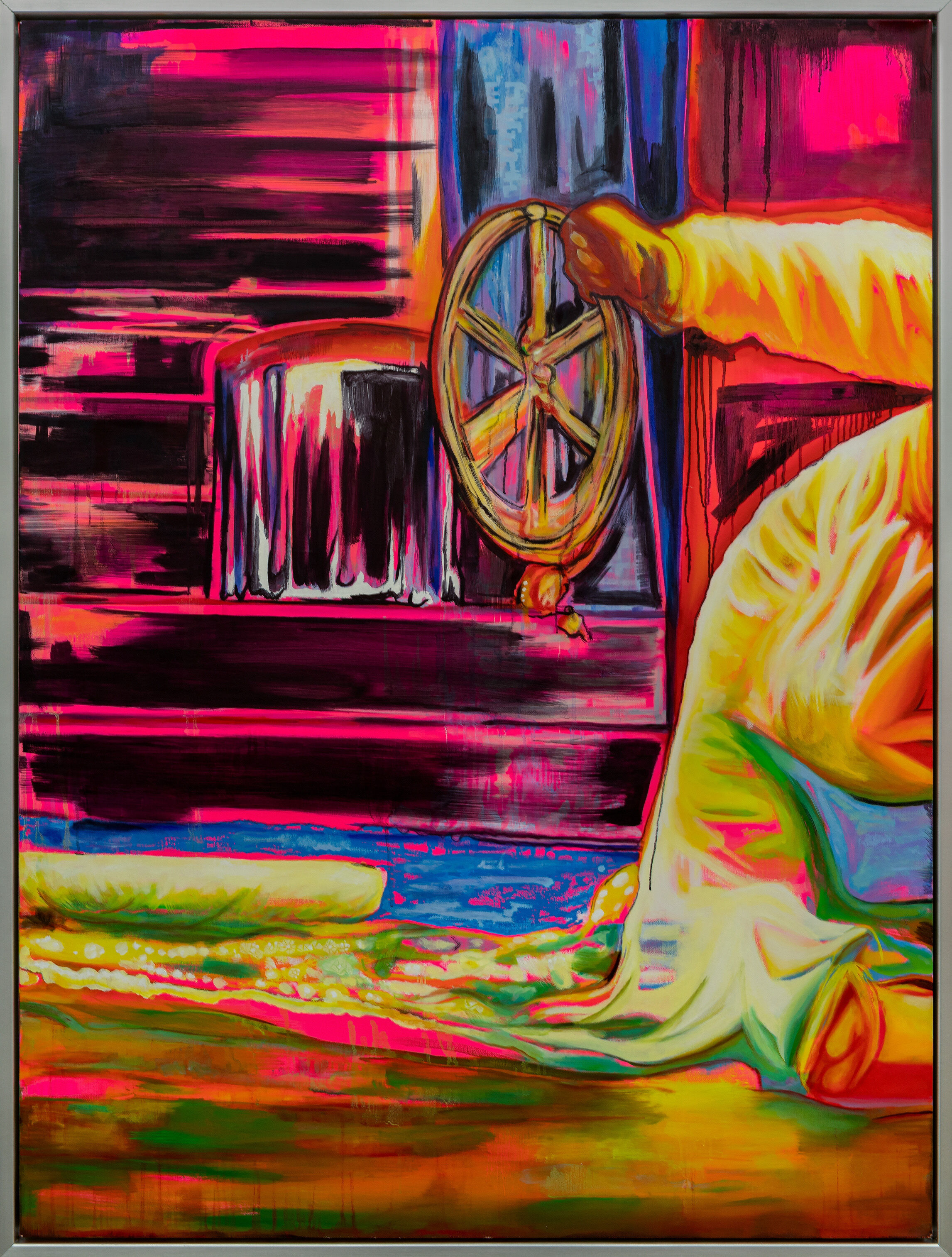The artwork appears to be either a digitally created or a hand-drawn painting with a distinctive abstract style. It features a vibrant yet dark palette, combining unexpected colors such as intense oranges, greens, magentas, electric blues, purples, and dark browns. The image depicts a partially seen figure—possibly a man—whose arm and back are visible as he grasps an orange-brown wheel. The figure is clad in a yellowish-golden robe embellished with accents of dark green, pink, and orange. The wheel, reminiscent of one found on a boat, is set against a backdrop that suggests the inside of a structure like a cabin or train, characterized by dark pink and maroon-colored walls. These walls might also feature a pink and white curtain. Behind the wheel, there is a window highlighted with dark blue, purple, and pink streaks. The floor beneath the figure is a chaotic blend of yellow, pink, green, and blue hues, evoking a tie-dye appearance. The overall composition is obscure and abstract, rich in color yet dark in tone, making it reminiscent of AI-generated art.